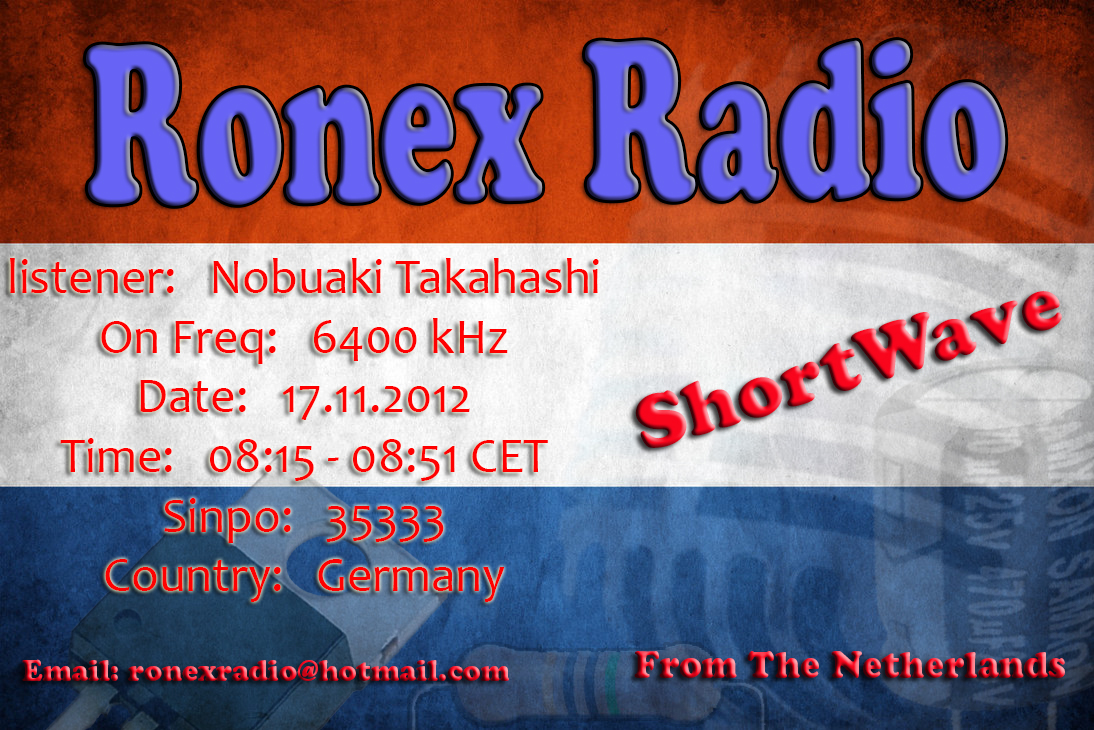The image is an advertisement designed with a flag-like background featuring three horizontal stripes: a red stripe at the top with the vibrant purple text "Ronix Radio," a white stripe in the middle with red text stating "listener Nobuaki Takahashi on frequency 6400 kilohertz, date 17-11-2012, time 8:15 to 8:51 CET," and a blue stripe at the bottom. At a 45-degree angle on the right side is the word "shortwave" in red text. In the blue stripe, it further reads "Sinpo 35333, country Germany," and "email Ronix Radio at hotmail.com from the Netherlands" in red text. An opaque background image of several microphones subtly enhances the advertisement.